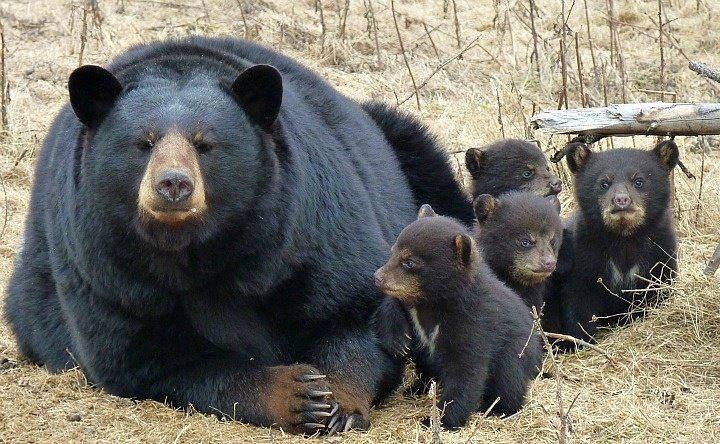This detailed image captures a serene woodland scene featuring a large black bear, presumed to be the mother, and her four cubs. The mother bear dominates the left side of the scene, lying on her stomach with her long claws touching each other. Her black fur is accented by a sandy brown snout and hints of brown at the tips of her paws. Her dark eyes gaze directly at the camera, and her rounded ears stand out, darker than the rest of her fur.

To the right of the mother bear are her four cubs, all similarly colored with black fur and sandy brown muzzles. Two of the cubs have distinctive light-colored 'V' or stripe markings on their chests. The cub nearest to the camera seems to find comfort with one paw resting on the mother bear's leg, while another cub looks directly at the camera. The two additional cubs are either partially obscured or gazing off in different directions, contributing to a sense of quiet activity.

The family is settled in an area covered with dead, straw-like grass and surrounded by sparse, dried vegetation, hinting at late autumn or early winter. A broken tree branch is positioned just above the head of the far-right cub, adding a rustic element to the scene. The overall setting, filled with muted browns and beiges of dry grass, twigs, and an occasional dead tree, highlights the contrasting dark fur of the bears and brings a sense of warmth and protection within this intimate family portrait.